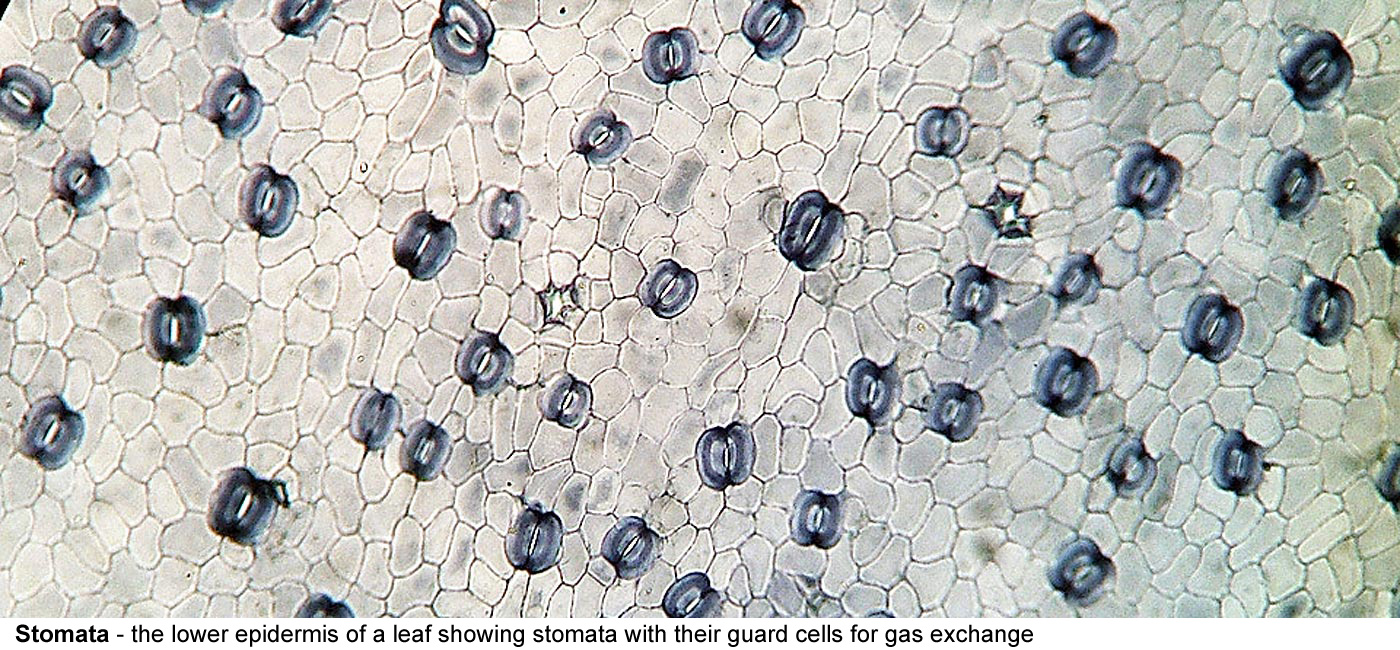The rectangular image closely resembles what you'd observe through a microscope, depicting an intricate scene evocative of snakeskin with its white and gray hues. Across this textured white-and-gray background are scattered dark navy blue, bean-shaped forms, resembling twin clamshells slightly parted to reveal a white central slit, akin to a pearl's glow within. These dark blue formations, identified as stomata, are uniformly detailed with a lighter central line, highlighting their role as gas exchange portals on the leaf's lower epidermis. The distribution of these stomata varies, with clusters more densely packed towards the image's right side and sparser towards the lower left. Below the image, a caption in bold black text reads, "Stomata," followed by a precise description, "The lower epidermis of a leaf showing stomata with their guard cells for gas exchange," providing a comprehensive context for this detailed cellular landscape.